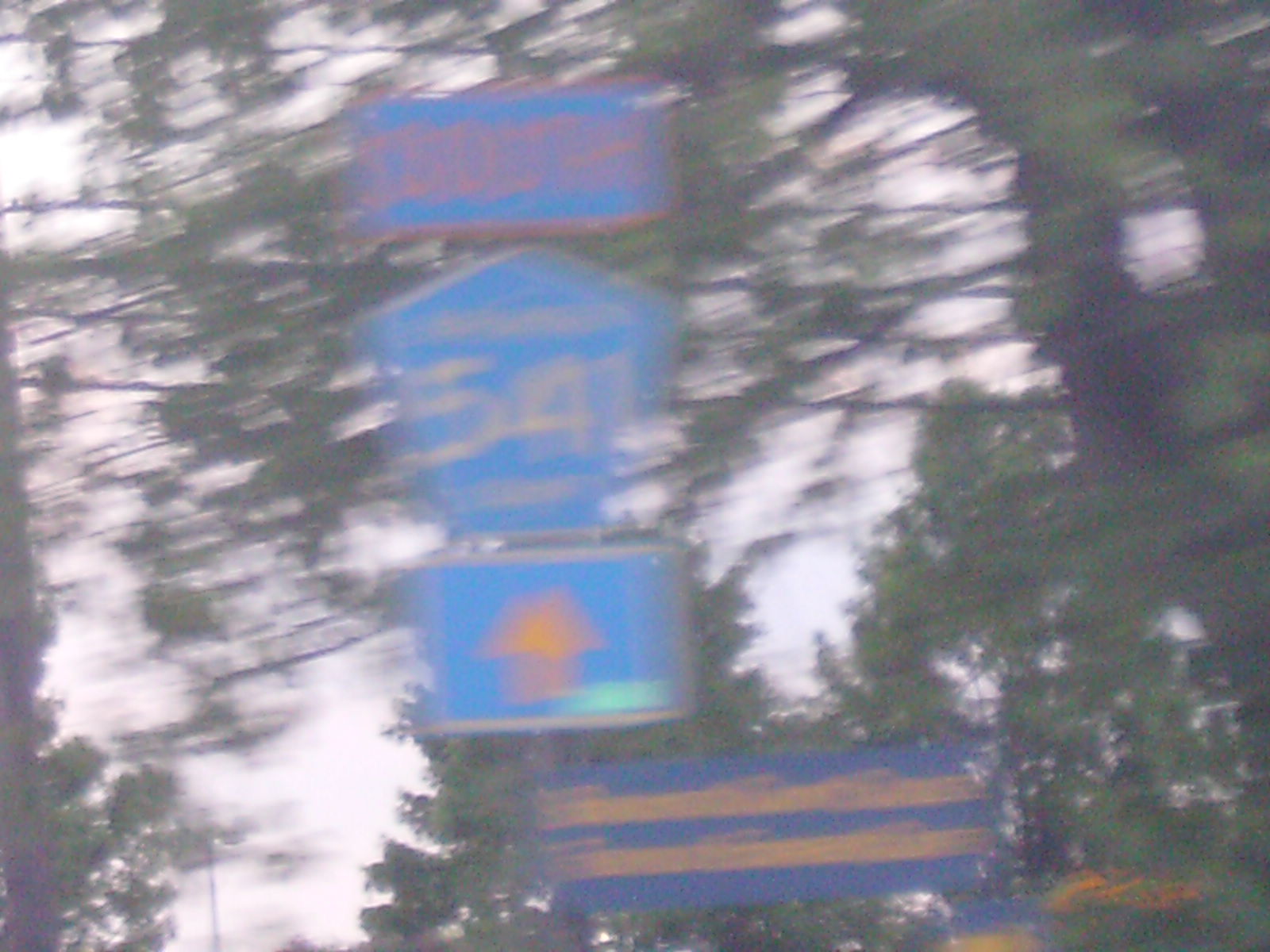This image depicts a very blurry and noisy photograph, likely taken from a moving car, capturing several street signs in front of a forested background filled with tree branches and green foliage against a gray, cloudy sky. In the foreground, a pole holds three blue signs: the top sign is a blue horizontal rectangle with red or orange text, possibly saying "South"; the middle sign is a blue pentagon clearly showing the number "54" in faded yellow letters, possibly indicating a route number; and the bottom sign, another blue horizontal rectangle, features an orange blob that might represent an arrow pointing upwards to indicate the direction straight ahead. Additionally, there is a separate elongated blue rectangle sign with yellow, unreadable text beside these. Electrical power wires are faintly visible among the trees, adding to the complexity of the scene.